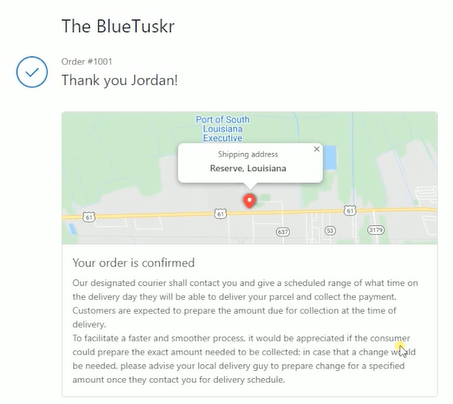**Detailed Caption:**

This image showcases an order confirmation from Blue Tusker, bearing the order number 1001, addressed to a customer named Jordan in Reserve, Louisiana. The confirmation message expresses gratitude for the order and specifies that the shipping address is located in Reserve, Louisiana. The message further confirms the order and outlines the delivery process, indicating that the designated courier will contact the customer with a delivery schedule. Upon delivery, the payment is to be collected, and the customer is advised to have the exact amount ready to ensure a smooth transaction. The message emphasizes that the courier may not have change, thus preparing the exact payment amount beforehand is crucial. Customers are reminded to confirm these details with the delivery person if necessary. The communication underscores the importance of readiness for both delivery and payment to facilitate an efficient process.